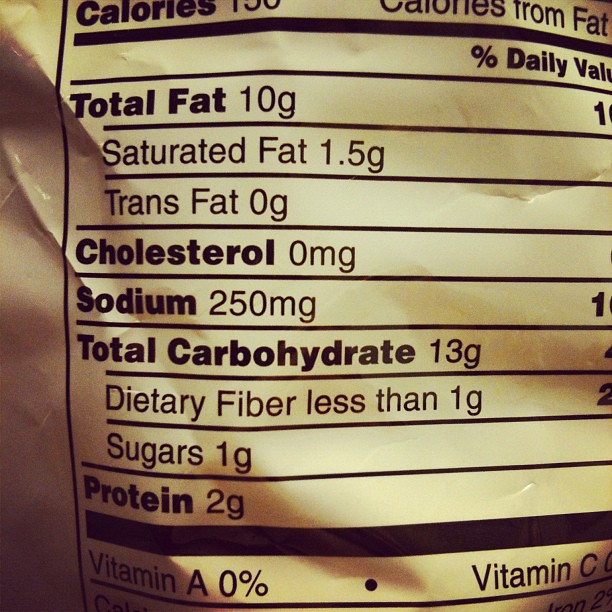This image is a close-up photograph of a nutritional label on a creamy yellow bag with wrinkles and creases, giving it a shiny appearance. The text, printed in black, is partially cut off at the top, missing the exact number of calories and calories from fat. The label lists the following in a clear, structured format: total fat 10 grams, saturated fat 1.5 grams, trans fat 0 grams, cholesterol 0 grams, sodium 250 milligrams, total carbohydrate 13 grams, dietary fiber less than 1 gram, sugars 1 gram, protein 2 grams. Vitamins A and C both have 0% daily value, and iron is listed at 2% in the bottom right corner. The background features tan shades in the shadowed areas, adding dimension to the creamy surface.